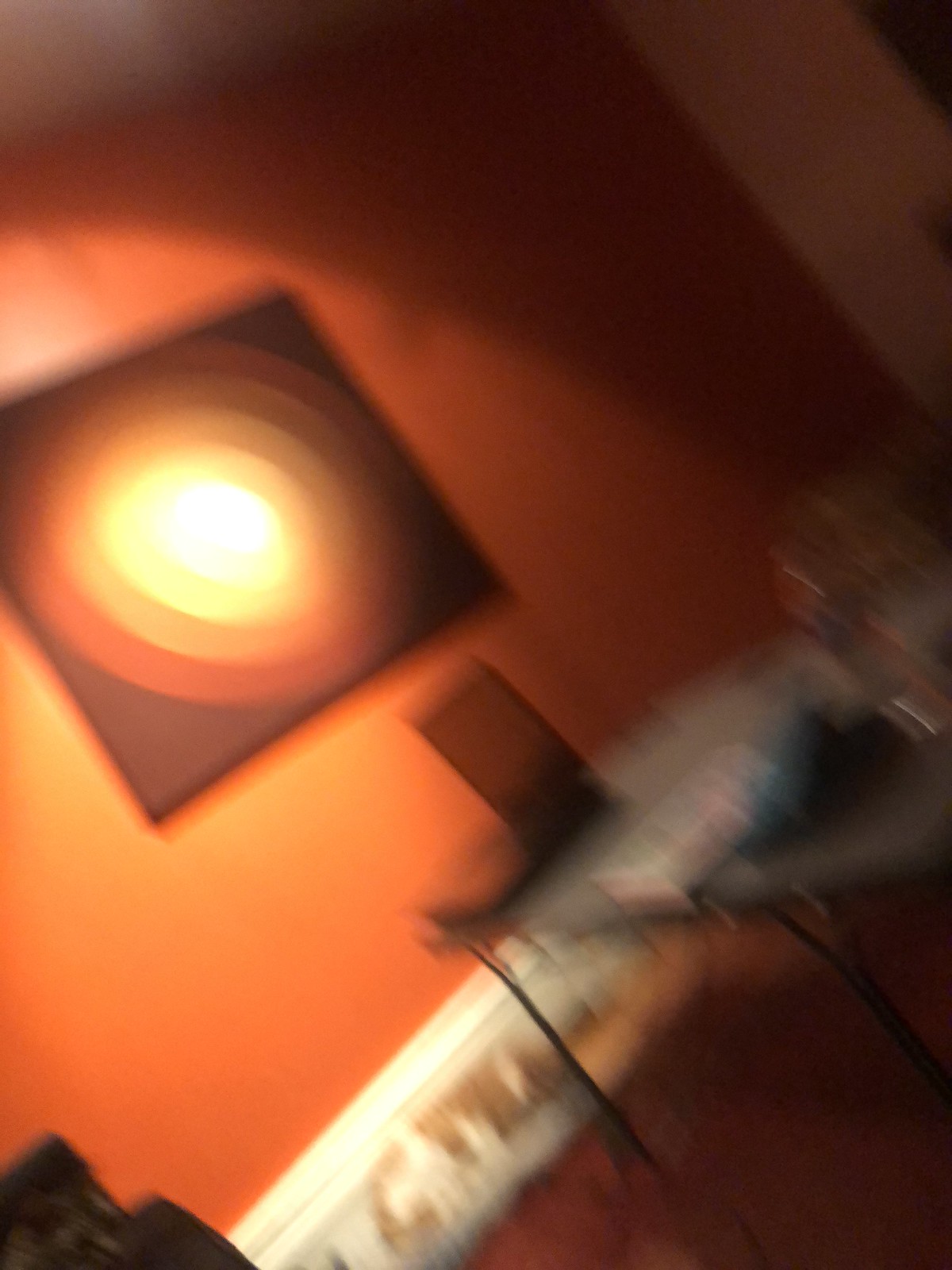The image depicts a somewhat blurry view of an office space, showcasing a corner of a room. The main wall in the center is a dark reddish-brown color, featuring a piece of artwork prominently. The artwork consists of concentric circles, starting with a bright yellow center, transitioning to light tan and various shades of brown, with a black background, all encased in a black frame. The floor is brown, and there's a strip of bright white trim at the base of the wall. A modern white table with black legs stands in the room, holding a black laptop and a white book among other indistinguishable objects. The adjacent wall, visible in the top right corner, is white, adding contrast to the darker tones in the main area.